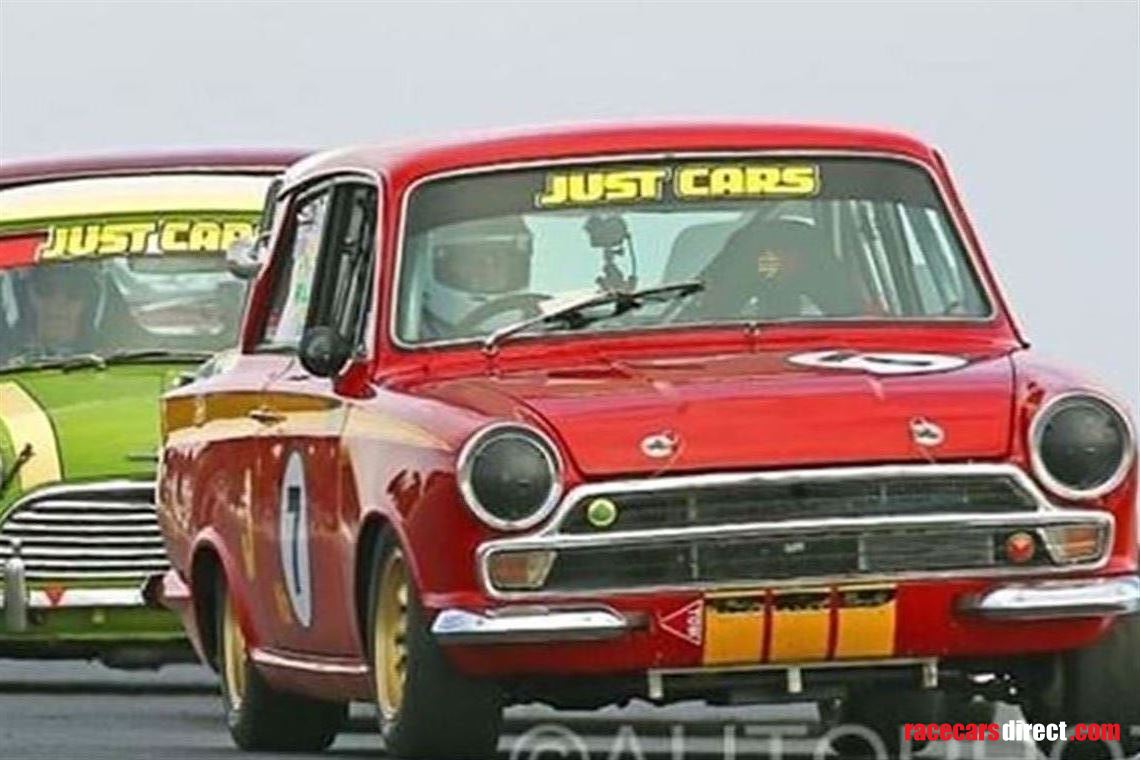The image captures a dynamic scene featuring two vintage race cars in motion. Dominating the frame is a bright red car, adorned with a prominent black number 7 encircled in white on the side door panel and hood. The car flaunts racing stripes along its bottom and has "Just Cars" emblazoned across the top of its windshield. The headlights are covered, with black round covers, while the split front bumper and shiny grille contribute to its classic aesthetic. Its gold wheels appear wider than typical for standard cars. The driver, seated on the right-hand side—typical of European vehicles—is seen wearing a white helmet. Trailing behind the red car is a lime green race car, also with "Just Cars" on the windshield, partially visible and featuring yellow stripes. In the bottom right corner of the image, the URL "racecarsdirect.com" is printed, where "racecars" is highlighted in red and "direct" in white.